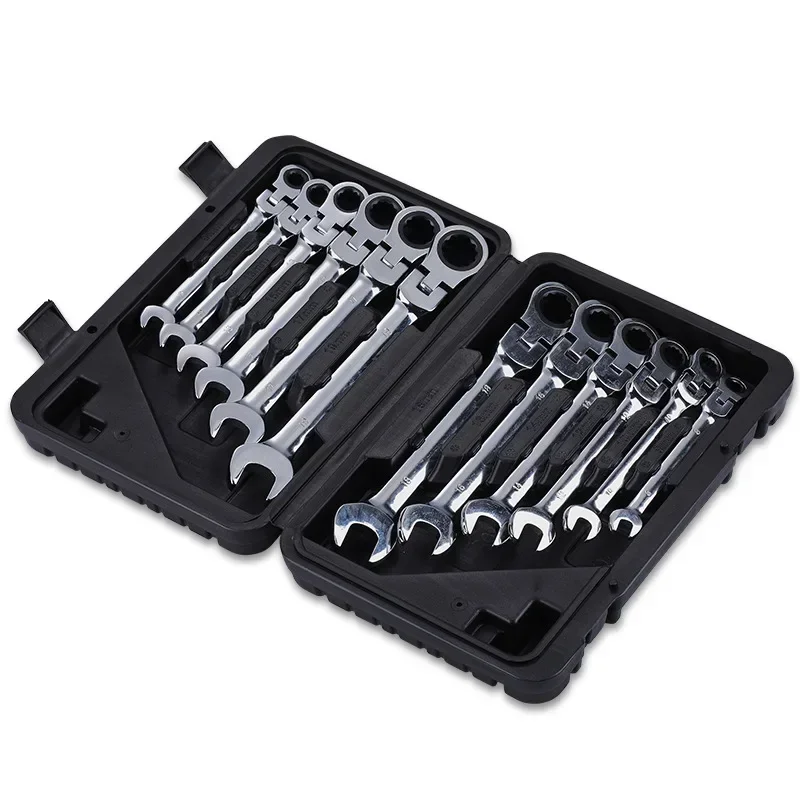This photograph features an advertisement-style image of a black toolbox with a white background, showcasing an organized wrench or ratchet set. The case opens like a book and contains a total of twelve silver-colored wrenches, each nestled in precisely cut depressions to keep them secure. The set is arranged with six wrenches on each side; on the left side, they range from smallest to largest, and on the right side, they transition from largest to smallest. Each wrench features a U-shaped open end resembling a horseshoe and a ratcheting circular end suitable for tightening or loosening bolts in a ratchet-style fashion. The toolbox, equipped with two latches to secure it when closed, is positioned slightly diagonally within the frame.